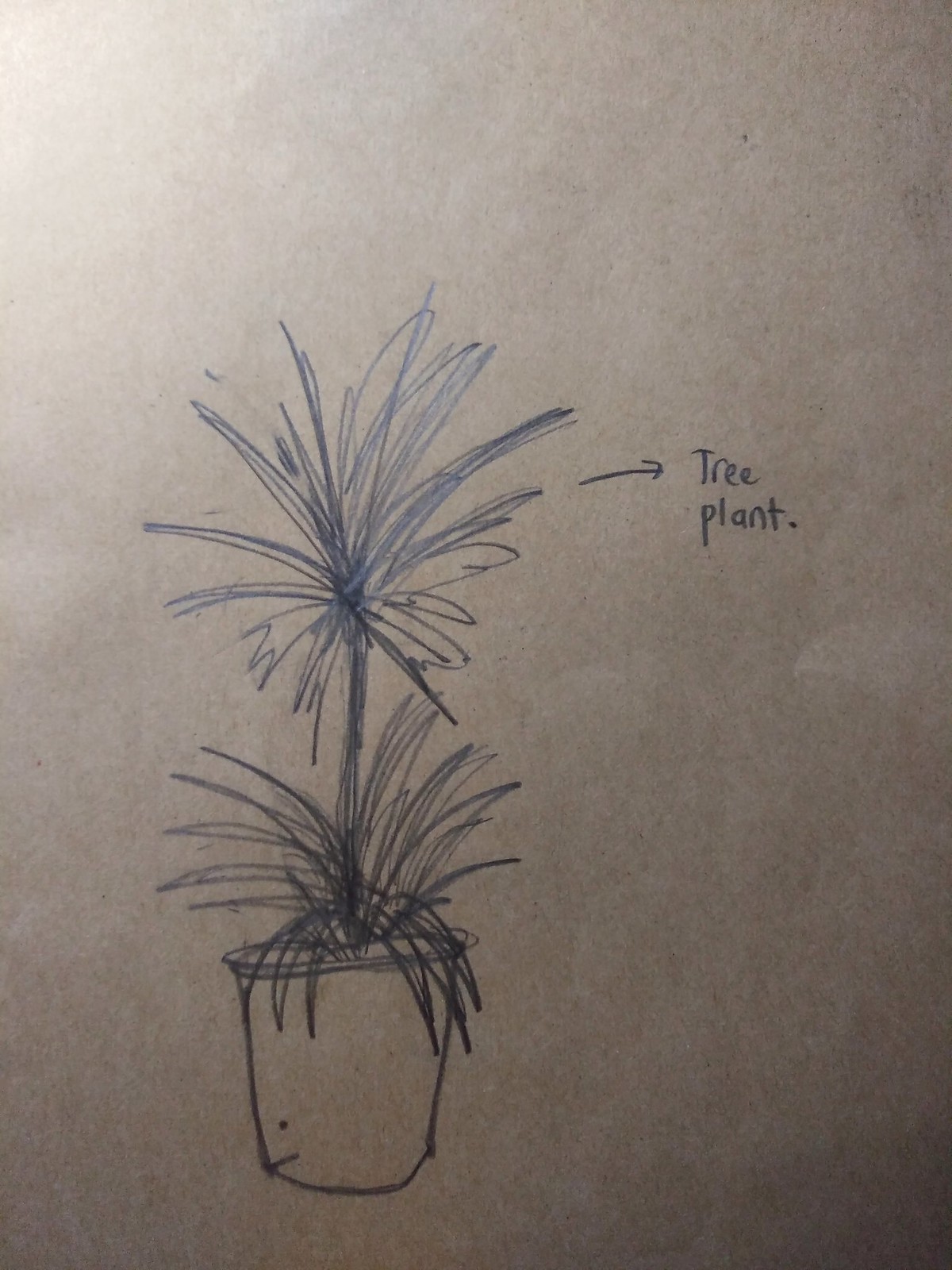This is a color photograph of a pencil sketch on slightly off-white A4 paper. The roughly drawn plant features a small pot with minimal detail, from which leaf-like lines protrude. At its base, the planter has some ambiguous elements that look like artistic detailing. From the small pot, a stem extends upward, supporting another tuft of foliage that suggests a flower. To the right of this upper tuft, an arrow points to a handwritten note in pencil that reads, "tree plant." The sketch is simple and lacks intricacy, capturing a basic and straightforward depiction of the subject.